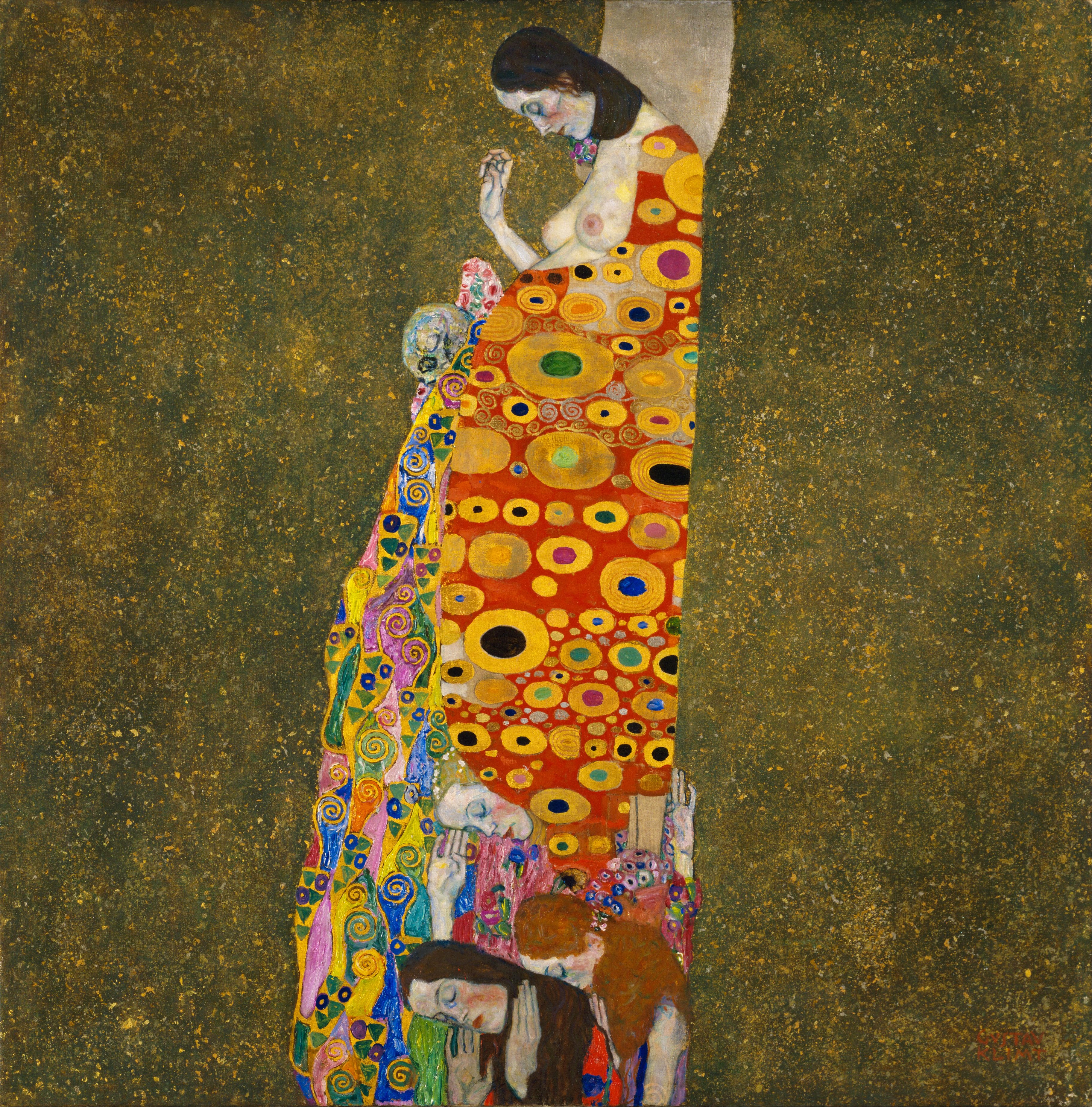This image features the painting "Hope II" by Gustav Klimt. The background is a dark, textured mix of yellow, brown, dark green, and black, resembling a speckled or sandstone surface. At the center stands a woman with dark, neck-length hair, slightly bowed head, and closed eyes, exuding a sense of introspection. She is depicted with a bare chest, and her right arm is gracefully raised. The woman is adorned in a richly patterned cloak predominantly red, embellished with gold and circles of varying colors such as black, blue, green, magenta, and orange, forming intricate geometric shapes.

The robe drapes elegantly down to the bottom of the image where three more female figures appear. These figures share similar postures to the central woman, with their heads bowed and hands raised. One has long brown hair, another has light brown hair, and the third features dark hair and a dark shirt. The artistic use of repeated patterns and the harmonious arrangement of colors create a mesmerizing and contemplative visual composition that is characteristic of Klimt's distinctive style.